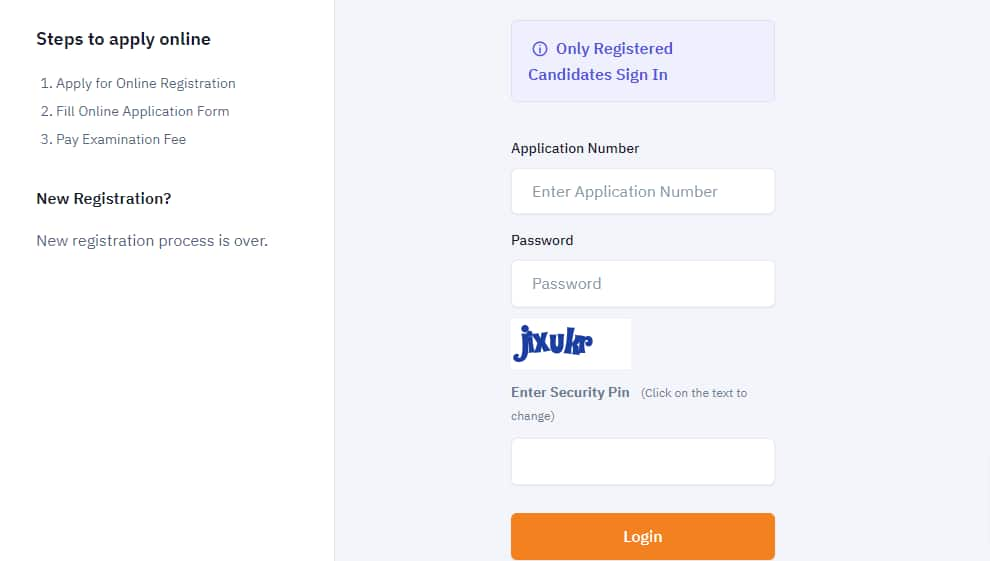This is a screenshot from a web page for candidate registration. At the top of the page, there's a message stating, "Only registered candidates sign in." Below this message, there's a field labeled "Application Number" with a white box where users can enter their application number. Following this are fields for "Password" and "Security Pin," each with corresponding boxes to input information. At the bottom of this section is an orange "Login" button.

On the left side of the page, three steps are listed under a section titled, "Steps to Apply." Beneath these steps is another section labeled "New Registration Window," accompanied by a message that reads, "New registration process is over."